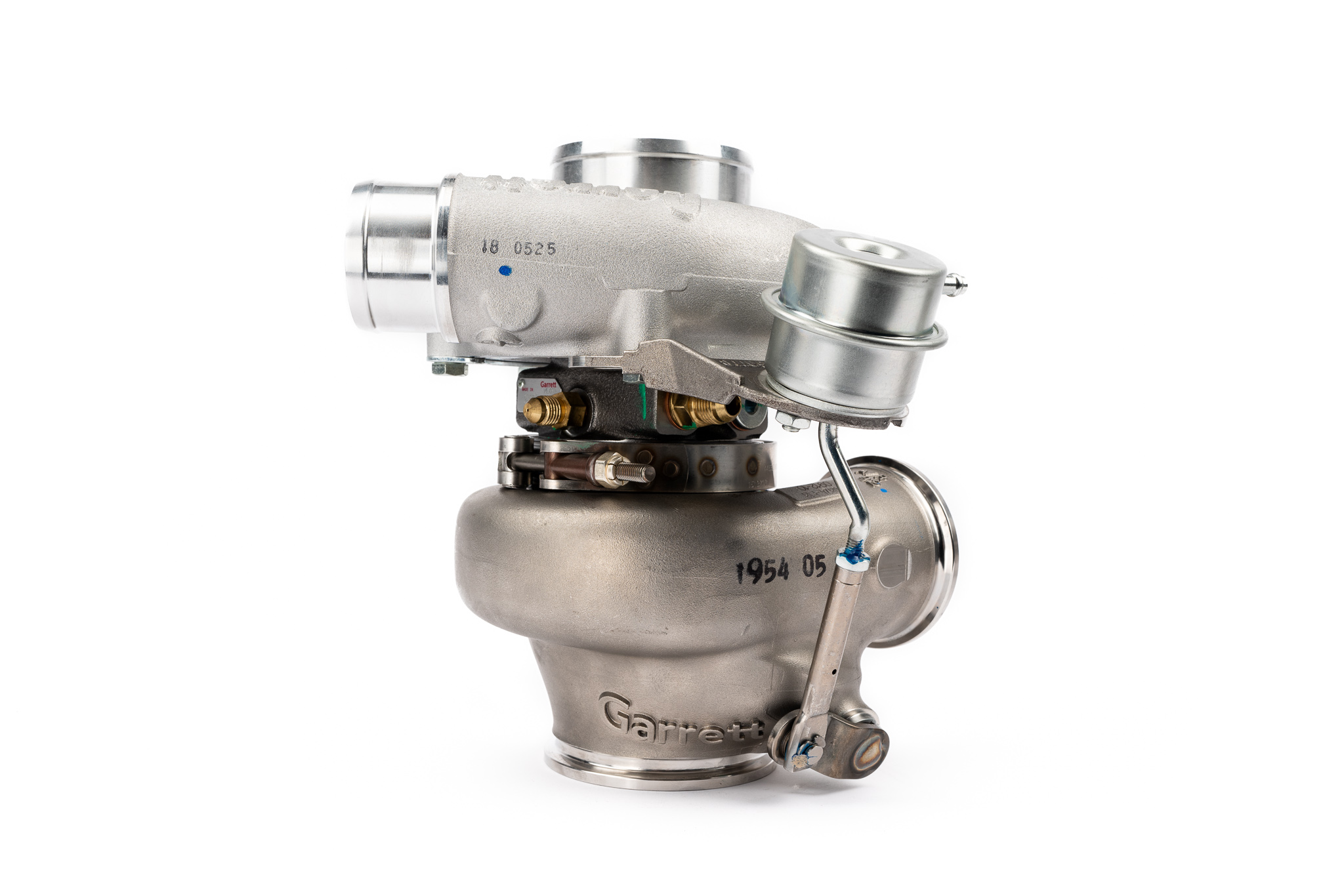The image depicts a motorized metal contraption, predominantly featuring the brand name "Garrett" emblazoned at the bottom. The device comprises two main cylindrical sections, one at the top and one at the bottom, held together by a central band with a tension bolt and metal bracket. The top section is silver and oblong in shape, possibly resembling a lens apparatus, and is connected to a double-stacked pipe that swirls downward. The bottom section is a warmer copper tone with smooth, rounded edges. The middle band, darker in color, displays the numbers "195405," while smaller digits, "180525," are inscribed on the top left. The intricate design highlights washers on the nuts, giving the assembly a complex yet precise engineering aesthetic. This detailed build is indicative of a sophisticated motor part, likely involving an intake and exhaust valve system.